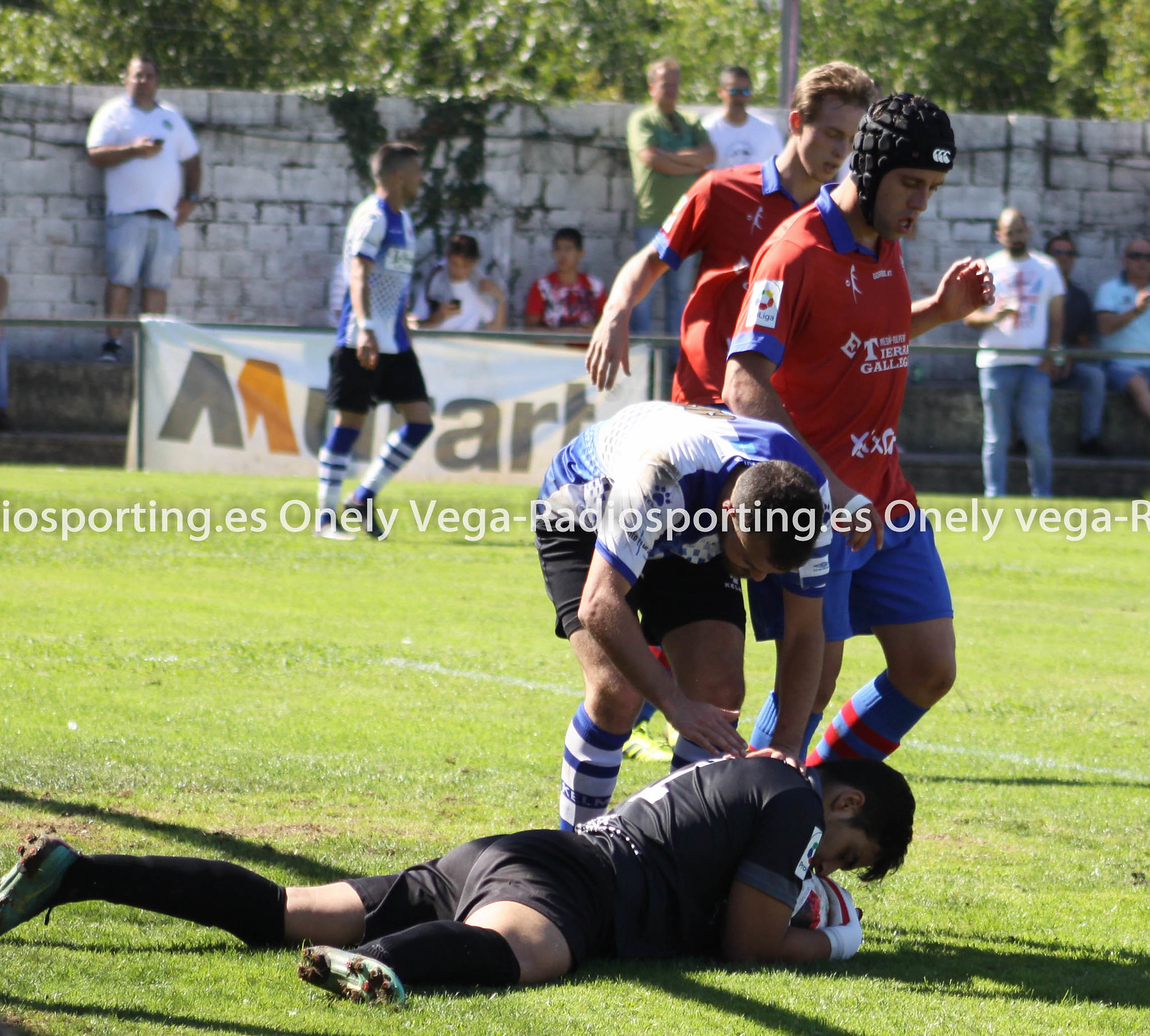In the foreground of the image, a soccer match is taking place during the daytime, evident from the shadows casting toward the right side. A player dressed in an all-black uniform with white writing, black knee socks, and white gloves is lying on the ground, clutching a soccer ball tightly to his chest. An opposing player in blue is crossing over him, patting the black-uniformed player on the back. Behind them, two players dressed in blue and red are walking toward the right side of the field. 

In the background, more details unfold: a man in blue and white with black shorts is seen walking to the right, in front of a gray gate lined with spectators. The spectators are standing against a white cement wall, watching intently. A white sign with a two-tone 'M' (gray on the left and gold on the right) as well as the text "OneLeagueVega-RadioSporting.es" can also be seen prominently displayed across the middle of the image. This scene captures a moment of dynamic athletic interaction and audience engagement in a sunlit soccer game.